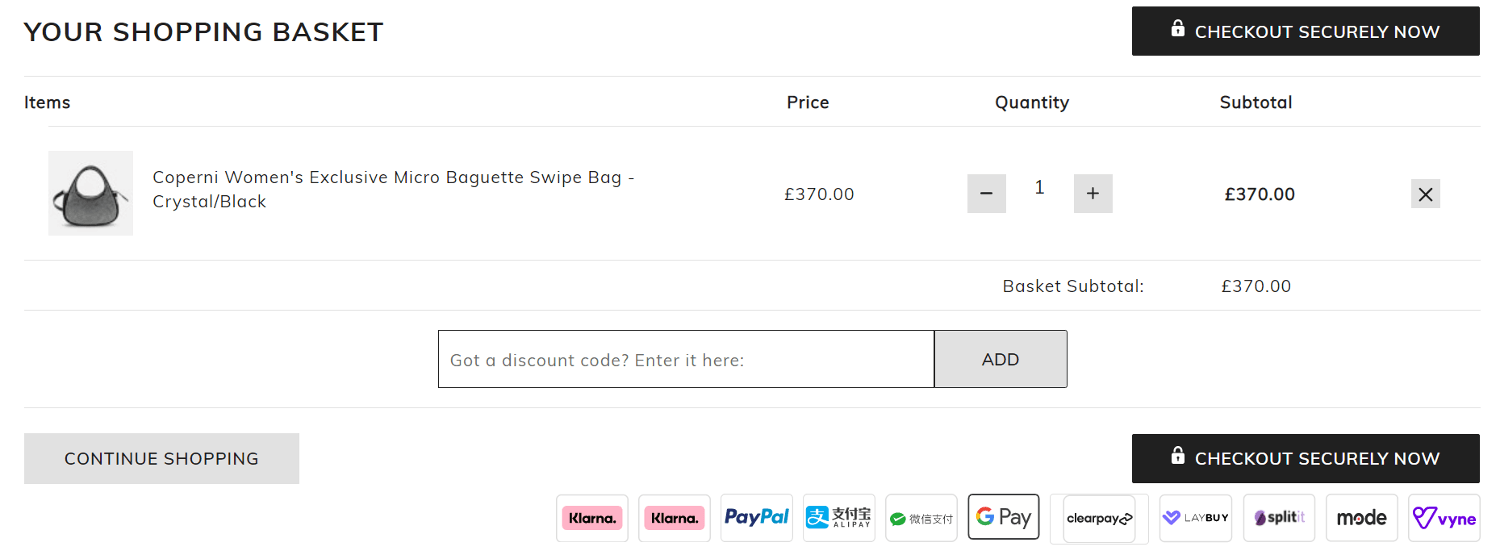Here is a detailed and cleaned-up caption for the given image:

---

The image portrays a shopping basket section of a website against a white background. At the top left corner, there is a black piece of text that reads "Your Shopping Basket." In the top right corner, a black button with white text and a white lock symbol says "Checkout Securely Now." Below, the page is divided into sections with headers for "Items," "Price," "Quantity," and "Subtotal."

Under the "Items" section, there is a detailed listing for a "Women's Exclusive Micro Baguette Swipe Bag Crystal in Black Color." To the right of this listing, the price is displayed as £370. The quantity is indicated as 1, making the subtotal also £370. Underneath these details, there is an area to enter a discount code. At the bottom section of the page, there are two buttons: "Continue Shopping" on the left and "Checkout Securely" on the right. Below these buttons, the accepted payment methods are displayed.